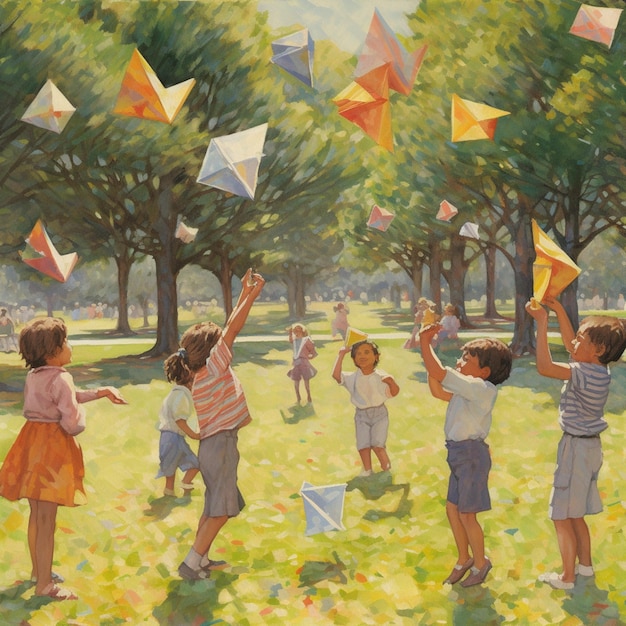This incredibly realistic drawing, which initially looks like a photograph, vividly captures a sunny summer day in a bustling park. In the foreground, a group of six children, both boys and girls, are joyfully throwing colorful paper airplanes into the air. The paper airplanes come in various shades including orange, blue, yellow, pink, and white, adding vibrant splashes of color to the scene. Among the children, a girl in an orange skirt with a long-sleeve white top and another wearing a striped orange, blue, and white t-shirt with gray shorts stand out. The boys are clad in blue jeans, white t-shirts, or khaki shorts paired with blue and white striped shirts. Surrounding the playful group is a lush green landscape with large trees and a concrete sidewalk or pathway cutting through the park. In the distance, more people can be seen enjoying the sunny day amidst the greenery, accentuating the lively and carefree atmosphere. The artist's attention to detail, from the children's attire to the textured leaves on the trees, enhances the realism of this captivating piece.